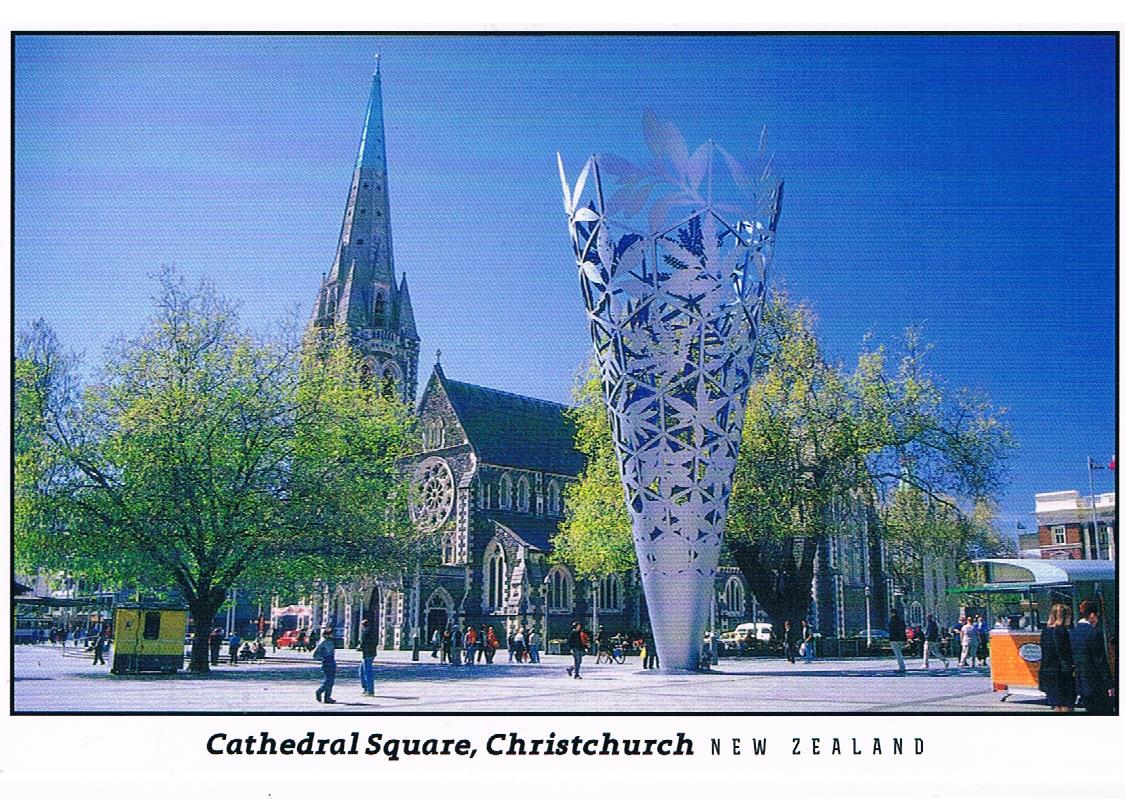This image, which resembles a postcard, depicts Cathedral Square in Christchurch, New Zealand, with the label "Cathedral Square, Christchurch, New Zealand" inscribed at the bottom in black letters. The photograph is set against a white background and is bordered by a thin black line. It captures a lively city square on a sunny, likely spring day, evident from the light green leaves on the two prominent, large trees. The square is bustling with pedestrians and has a few cars parked in the distance.

Central to the square is a striking large metal sculpture, an inverted cone shape intricately woven with silver metal leaves. Beyond the sculpture stands an ornate gray stone cathedral, distinguished by its tall, pointed tower and white-outlined stained glass windows. The beautiful blue sky frames the scene, and various stands can be seen, including a noticeable yellow and orange stand. The overall ambiance suggests a vibrant public space, frequented by both tourists and locals. The background features light grey and brown paving, with overhead wires crossing between buildings, adding to the urban charm of Cathedral Square.